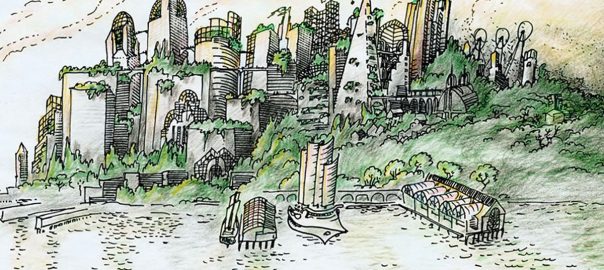This illustration, reminiscent of the art styles of "Rocko's Modern Life" and "Ren & Stimpy," depicts a vibrant, cartoonish city situated along a coastline. The city is set against a hill and features a variety of distinctive, stylized buildings, all heavily adorned with lush greenery, almost as if nature has overrun the structures. Among the eclectic architecture, notable features include a tall pyramid-like structure, a greenhouse on the water, and a collection of brutalist towers. The scene, observed from the water which appears a speckled white rather than blue, also includes multiple piers and docks, some with awnings and sailboats. The overall ambiance is a blend of futuristic and fantastical, presenting a whimsical, lively urban area flourishing with green spaces and creativity, yet devoid of any people.